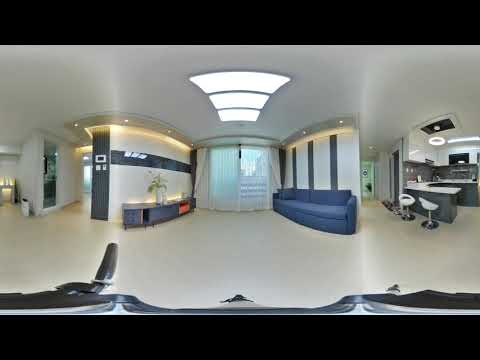This image, likely a 360-degree photo, showcases an immaculate and sophisticated indoor space that might be a modern apartment or possibly an upscale office, spa, or exercise area. The room features an elegant aesthetic with white floors, walls, and ceilings. Overhead, there are centrally-located, large square-shaped lights that resemble fluorescent lighting, progressively increasing in size.

Dominating the center of the image is a double sliding glass door adorned with white translucent drapes. To the right of the doors, a comfortable blue loveseat sits adjacent to navy blue or dark grey wall stripes. In front of it is a sleek blue TV stand or credenza, though no television is mounted on it.

On the far right of the image, the space transitions into a contemporary kitchen area, which includes black counters contrasted with white countertops and curved white bar stools. The kitchen is further accented by a black tile backsplash and white upper cabinets. A hallway, likely leading to other rooms, is visible from the kitchen.

Additionally, on the left side of the image, there is a garbage can and another hallway, implying an extended layout. A mirror on the left wall increases the room's spacious feel. The scene is devoid of people and text, highlighting its pristine and serene environment, which could easily be suited for relaxation, work, or light exercise such as yoga.